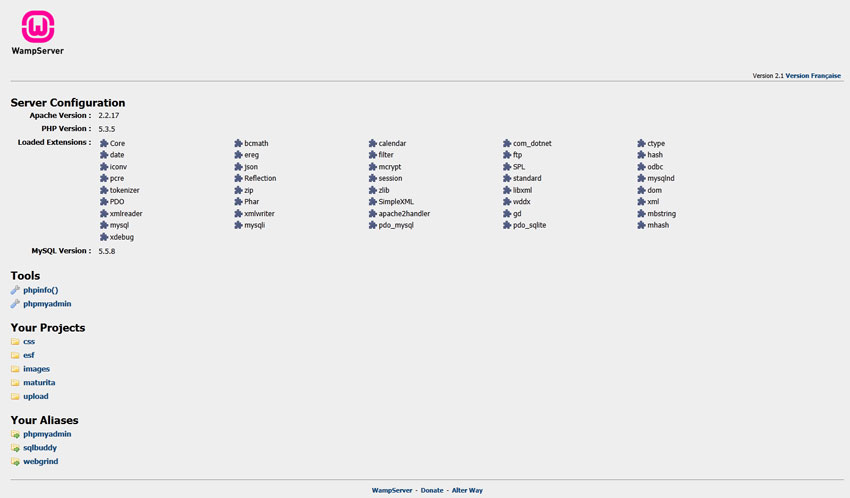This cropped screenshot displays the WAMP Server, a web development platform used on Windows for creating web applications in various programming languages. The background is a muted grey, and the WAMP logo is prominently positioned on the top left of the page. The version information, "2.1," is subtly printed in small black letters near the top right, slightly offset towards the bottom of the header section.

A grey bar horizontally divides the header from the main body of the page, providing a clear separation between the sections. Just beneath this bar on the left side, the text "Server Configuration" is presented in bold black letters. This section details the Apache version, PHP version, and the loaded extensions.

Below this, five distinct rows of extensions are displayed, with each row containing eight extensions. These are listed horizontally across the page in a neat, organized manner.

Following the extensions section is the "Tools" section, which lists two available tools. Beneath the tools, the "Your Projects" section is featured, including a folder subsection that likely contains user-specific projects. At the bottom of the left column, under the "Your Aliases" section, three login options are shown.

The overall layout is clean and organized, allowing users to quickly access server configurations, tools, projects, and login options within the WAMP Server interface.